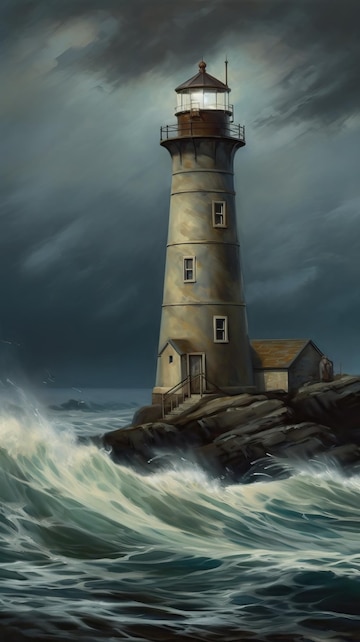The painting depicts a stormy maritime scene centered around a lighthouse standing resiliently on a rocky outcropping amidst tumultuous, bluish-green waves. Dark gray and black storm clouds dominate the sky, swirling from the top right corner to the bottom left, indicating a relentless downpour. The lighthouse itself, constructed of a weathered, gray metal with patches of brown and beige hues, features a distinct patina and an uneven coat of paint, evidencing its battle against the harsh elements. It has three small windows situated at different tiers along its vertical shaft and a doorway at the base, accessible via a set of stairs leading down to the treacherous rocks. At the pinnacle, a red-tinted top encircles the light chamber, from which bright beams cut through the stormy gloom, casting a faint illumination on the chaotic waters below. A railing encircles the light chamber, adding to the structure's intricate design. Behind the lighthouse, there is a modest house-like structure with an A-frame roof, adding a sense of scale and context to the scene. The crashing waves at the base of the lighthouse create a dramatic white spray, emphasizing the ferocity of the storm.